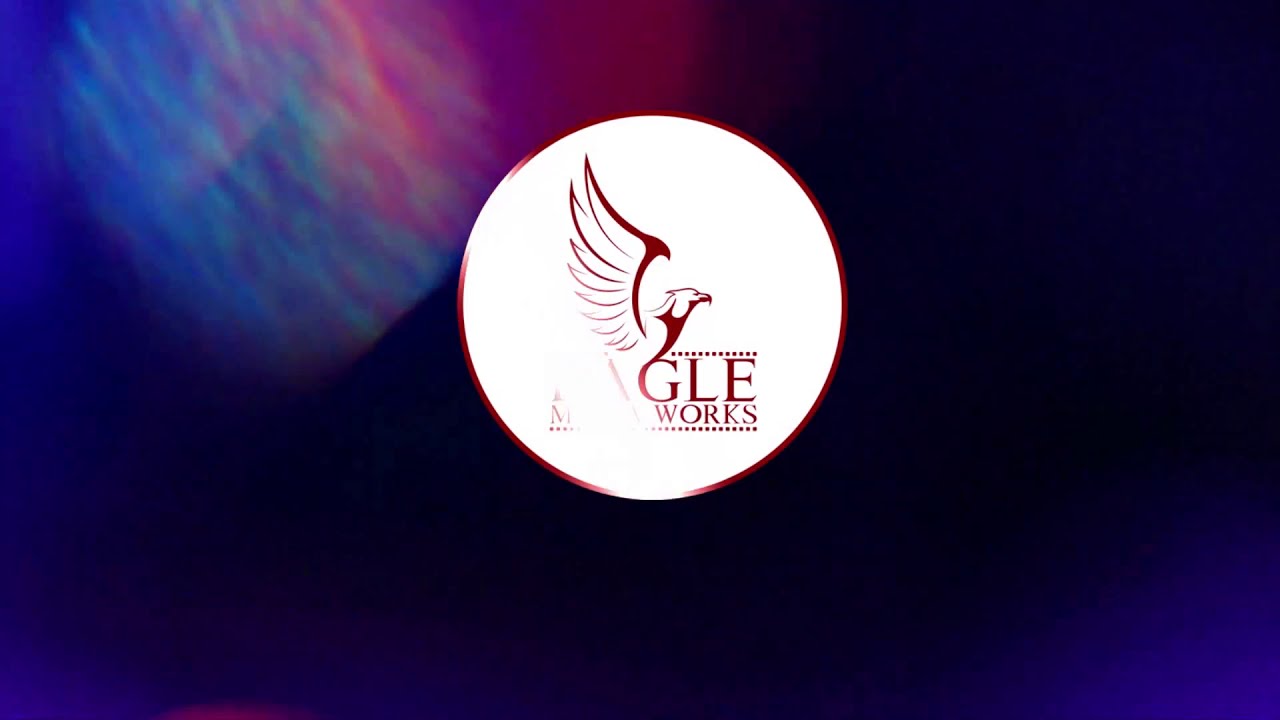The image, likely an advertisement or promotional graphic for a business or company, features a richly detailed, abstract background with multiple colors. The predominant shades are dark navy blue and deep purple, with a lighter shade of purple in the lower right corner and a blend of maroon, blue, and purple in the upper left corner. Central to the image is a white, or off-white, circular disk bordered by a maroon ring. Inside this disk, there is a maroon and white logo depicting a griffin-like creature with the head and wings of an eagle and the body of a mammal.

Due to a faded line running down from the eagle, only part of the text is visible. The text, in capital letters and a rich reddish color, is split into two lines: the first line reads "GLE" and the second line reads "WORKS." The design elements, including the background's abstract and multicolored sections and the reddish maroon accents of the logo and text, create a striking and visually engaging advertisement.